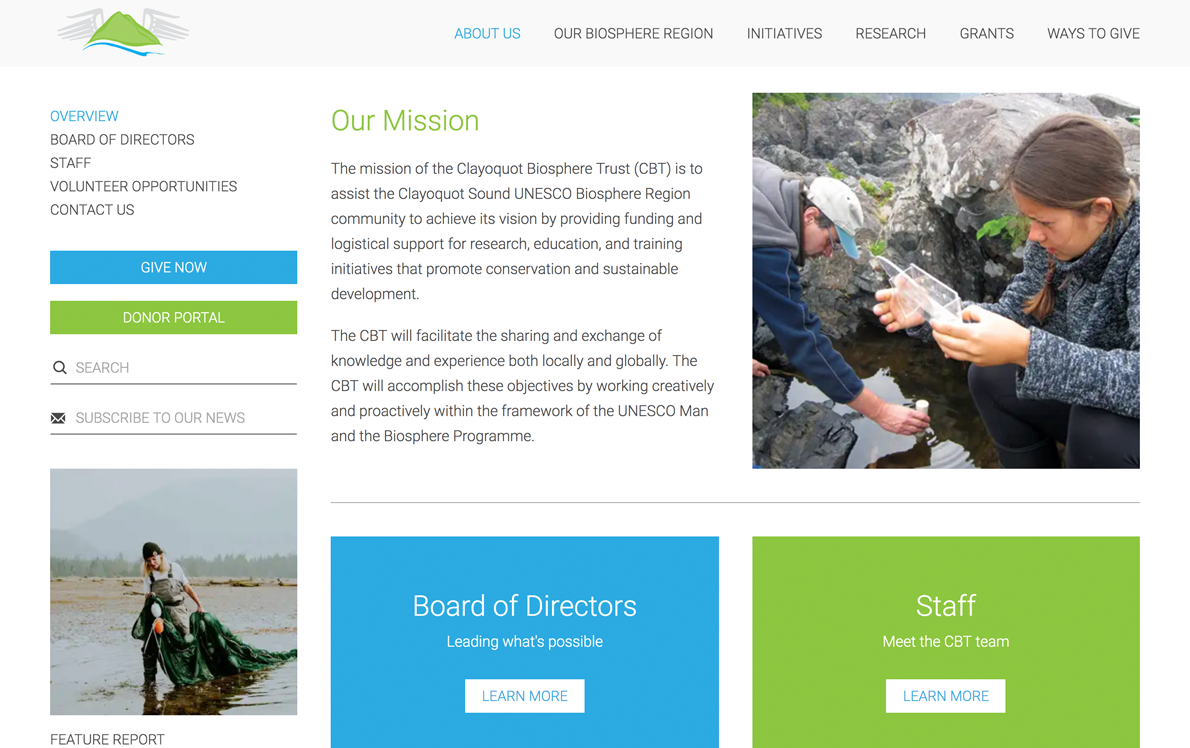Screenshot of the "About Us" page for the Clayoquot Biosphere Trust (CBT). The header features the CBT logo on the left—a green mountain with grey mountain shapes in the background—and navigation links reading: About Us, Our Biosphere Region, Initiatives, Research, Grants, and Ways to Give.

The page is divided into two main sections. On the left, there is a menu including links for Overview, Board of Directors, Staff, Volunteer Opportunities, and Contact Us. Below these links are two buttons: a blue button labeled "Give Now" and a green button labeled "Donor Portal."

There are two images on the page. In the bottom left corner, a photograph shows an individual dragging nets across a sandy shore. In the top right corner, another photograph depicts two people examining samples from water collected between rocks.

A mission statement is prominently displayed in the center of the page. Beneath this, there are two information boxes: a blue box highlighting the Board of Directors with the text "Leading What's Possible" and a green "Learn More" button, and a green box introducing the Staff with the text "Meet the CBT Team" and another "Learn More" button.